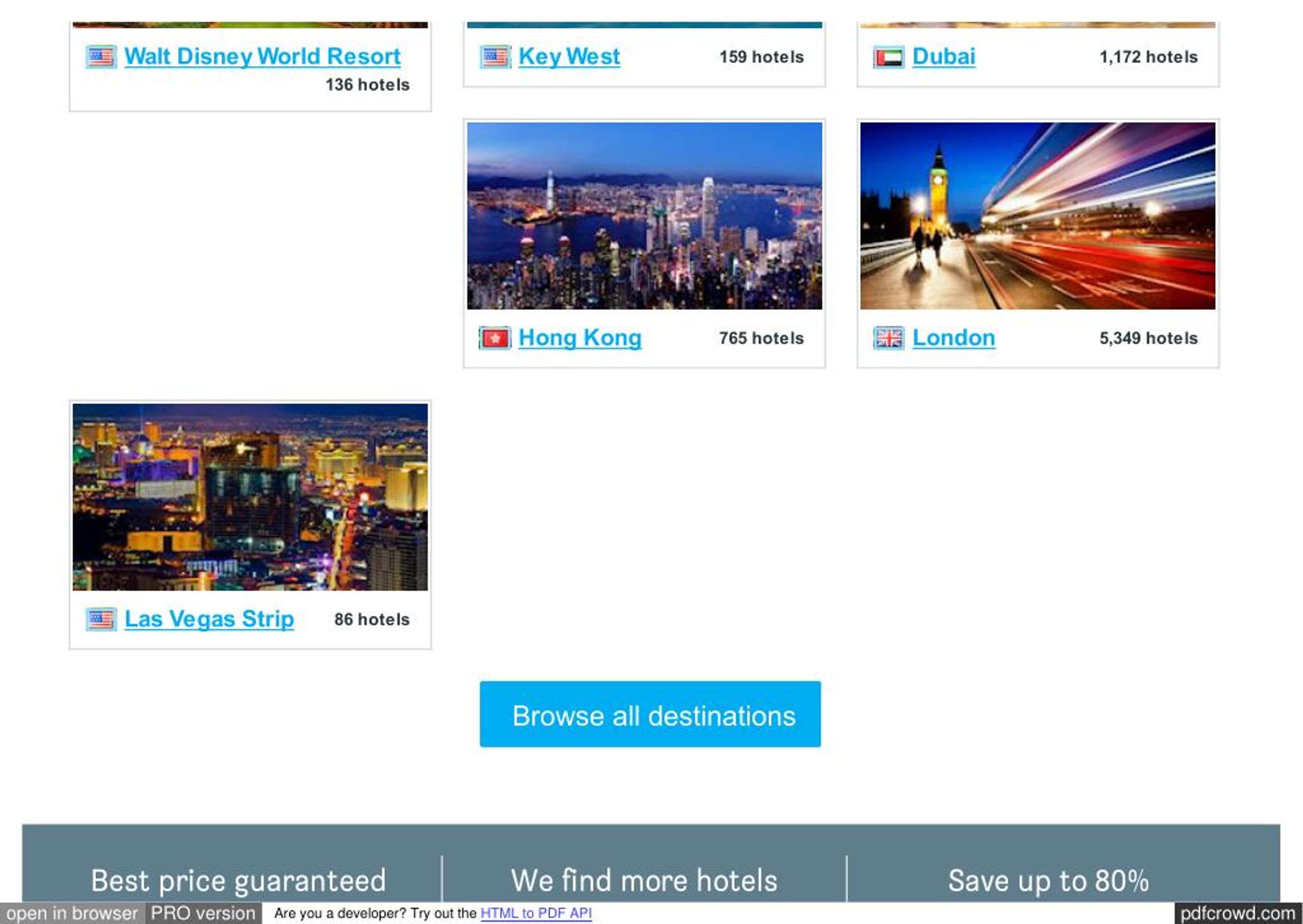This is a screenshot from a travel website or app, showcasing various travel destinations and related information. The interface is divided into three main columns, each featuring different travel destinations. However, due to some layout issues, the content is not fully visible. 

At the top, there are several destination options, but only the bottom few pixels of their thumbnails are visible. Below these thumbnails are links to the respective destinations:
1. **Walt Disney World Resort** (USA) with 136 hotels.
2. **Key West** (USA) with 159 hotels.
3. **Dubai** (UAE) with 1172 hotels.

However, the Walt Disney World Resort link is causing layout issues due to its length, which pushes the number of hotels to the next line, disrupting the alignment.

Further down, the affected layout continues:
1. **Hong Kong** with 765 hotels.
2. **London** with 5349 hotels.
3. **Las Vegas Strip** with 86 hotels.
4. An option to **Browse All Destinations**.

At the bottom of the screenshot, there's a gray panel with three options in a triple-column layout:
1. **Best Price Guarantee**.
2. **We Find More Hotels**.
3. **Save Up to 80%**.

The page design needs adjustments, particularly more padding around the options to prevent text overflow and misalignment.